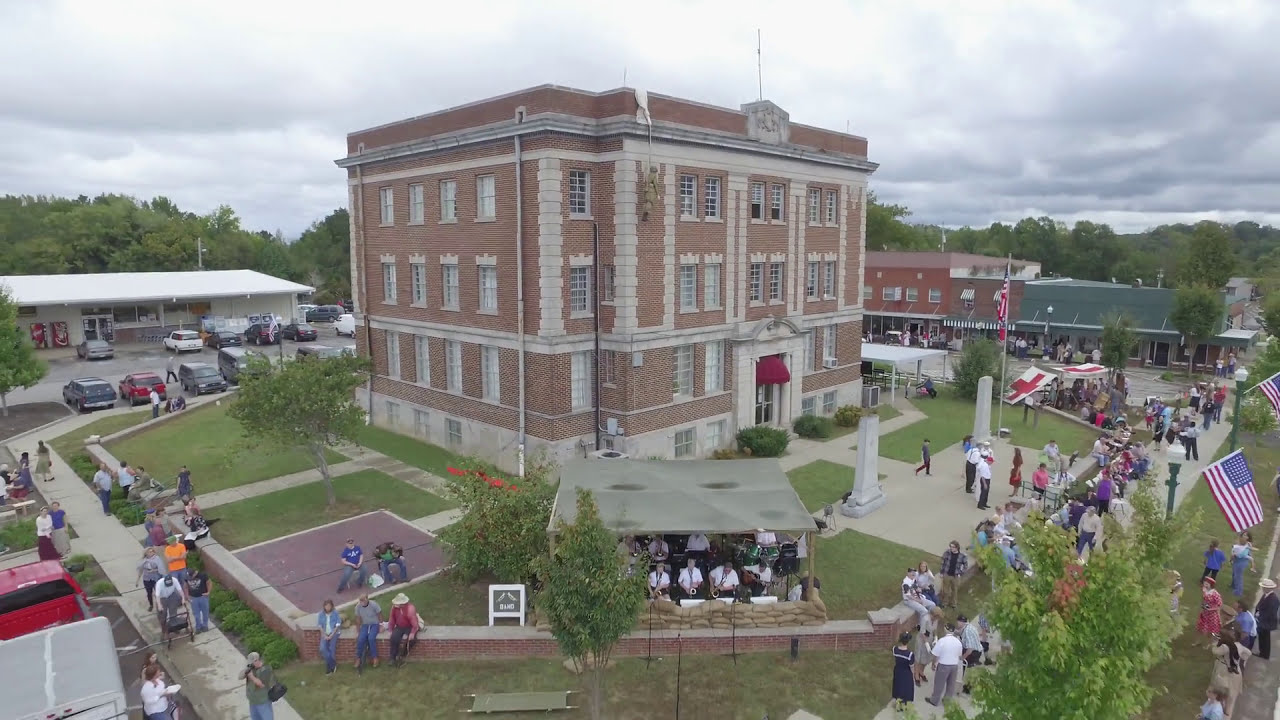The image depicts a bustling town square centered around a prominent, light brown, three-story building made of stone or brick with white trim around the windows and corners. The top of the building displays a traditional orange brick hue. An ottoman in front of the building’s entrance stands out in red or maroon. The sky above is overcast with white clouds, although patches of blue peek through on the left and right sides. A backdrop of tree lines, tall green trees with brown trunks, frames the scene.

To the left of the main building is a white, flat-roofed structure while on the right side, a series of buildings in brown and green hues can be observed. The building itself is encircled by a brick ledge that matches its tan color, with gray sidewalks wrapping around it and extending into the town square. Adding to the vibrant atmosphere, crowds of people, some wearing white shirts and dark pants, appear to be gathered for a festival or event. Among them, a group of musicians playing gold-colored instruments such as trumpets and trombones can be seen.

Numerous cars, in shades of red, blue, white, gray, and black, are parked around the area. In the far left of the image, near the white building, Coca-Cola machines, distinct in their red and white branding, stand out. There are American flags prominently displayed in front of the main building, along with green light poles and two gray cement posts. Two small white and red signs, one bearing a cross, are also visible. The scene exudes a communal and festive vibe, set in an inviting outdoor space with lush, green squares of grass dotting the landscape.